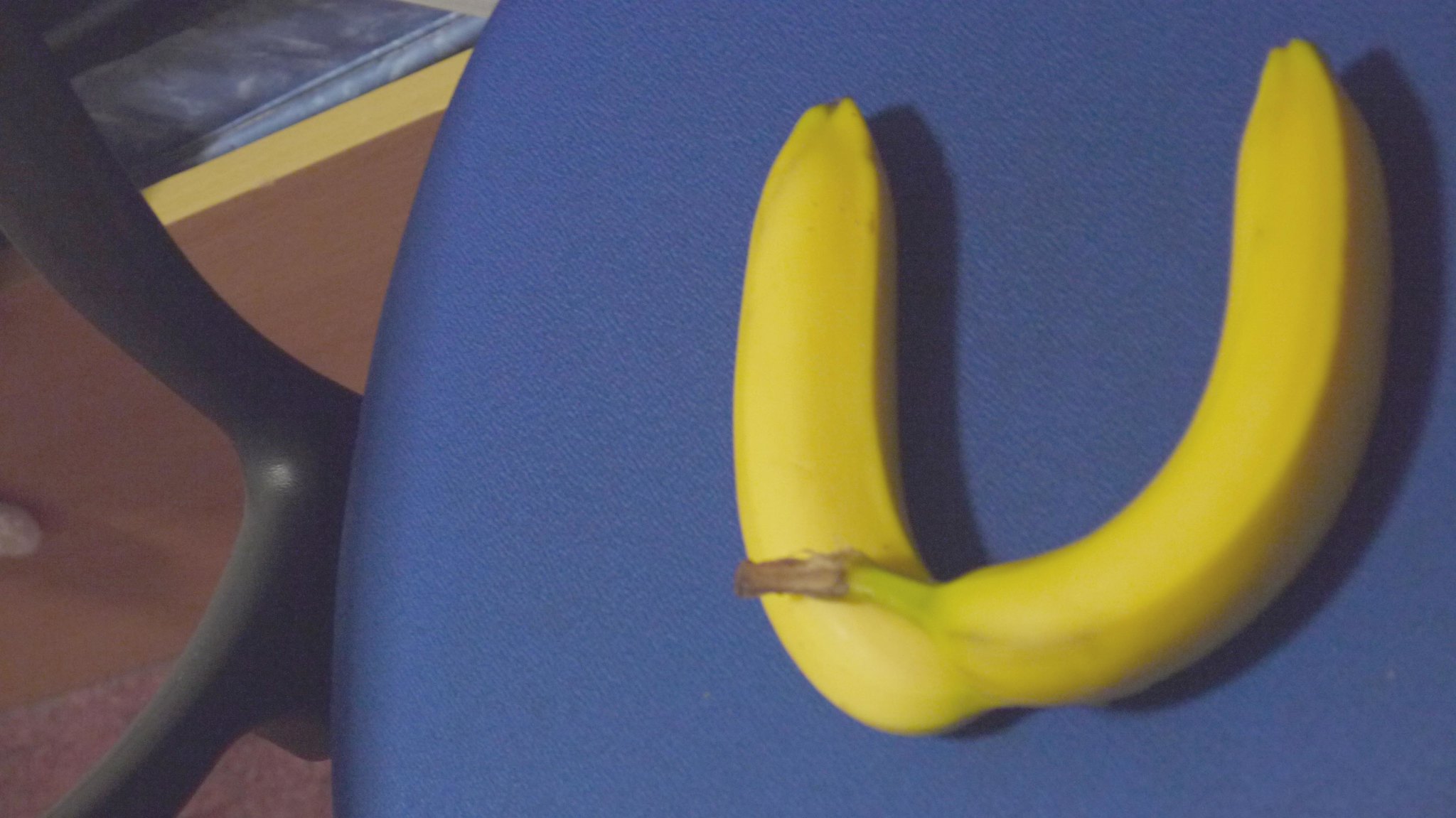This photograph, taken from an aerial perspective at a slightly tilted angle, features a table draped in a blue tablecloth. On the table, two bright yellow bananas are positioned in such a way that they form the shape of a letter "U," their stems overlapping. The bold yellow hue of the bananas contrasts sharply with the blue tablecloth. To the right of the table, a dark brown chair is tucked in neatly. In the background, beyond the table, there appears to be a partially visible drawer that likely belongs to a taller chest of drawers outside the frame. The floor is carpeted in a rich red or burgundy color. Notably, the bananas cast a distinct shadow on the tablecloth behind them, creating an intriguing W-shaped pattern that adds an artistic quality to the image.